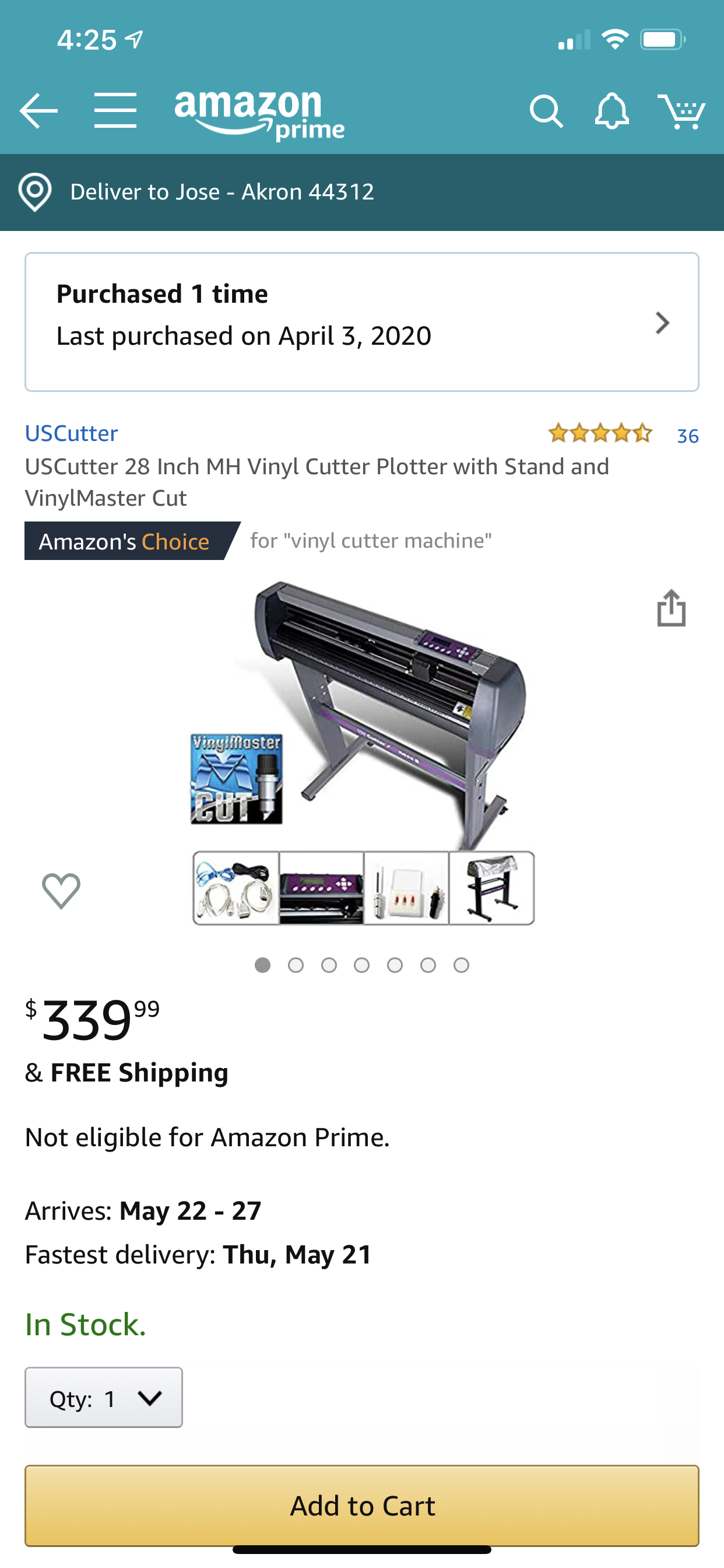Here is a detailed and cleaned-up caption for the described image:

---

Screenshot of the Amazon Prime interface at 4:25 PM, with the Wi-Fi icon showing two bars and a battery level at 95%. The interface features a turquoise blue Amazon Prime logo, a dropdown menu icon, and a search magnifying glass alongside a bell and a shopping cart. An arrow points to a notification that reads "Delivered to Jose, Akron 44312," with details indicating the item was last purchased on April 3, 2020.

Highlighted in blue is "U.S. Cutter," and below, in black text, it reads "U.S. Cutter 28-inch MH vinyl cutter plotter with stand and vinyl master cut." The product has received a rating of four and a half stars from 36 reviews and is marked as "Amazon's Choice" for vinyl cutter machines. The term "vinyl cutter machine" is in gray text.

A picture of the vinyl cutter device is displayed, with a heart icon on the left for adding the item to a favorites list. The price is listed as $339.99 with free shipping, though it is not eligible for Amazon Prime delivery. The estimated arrival dates range from May 22nd to May 27th, with the fastest delivery available by Thursday, May 21st. The item is in stock, indicated in green, and features a quantity dropdown menu. There is a gold "Add to Cart" button with black text at the bottom.